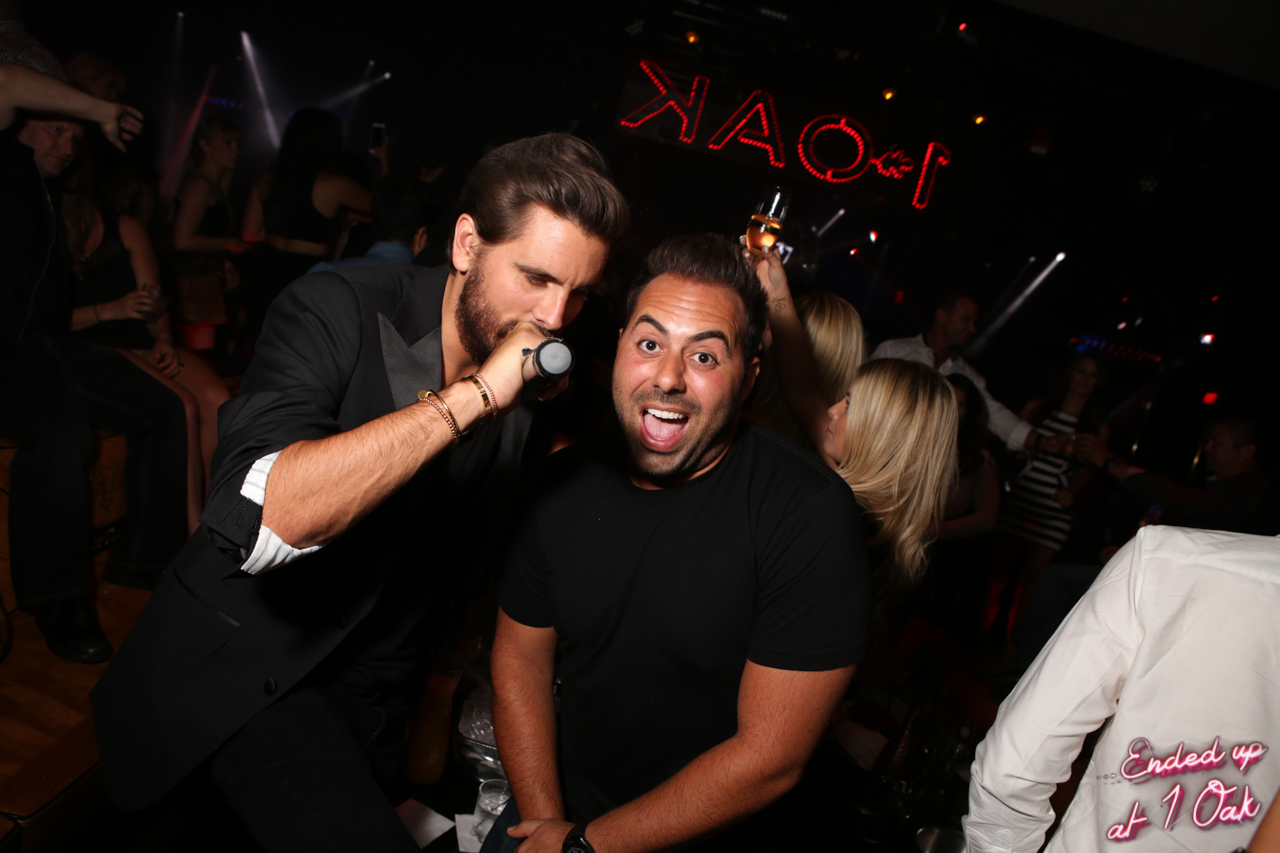In this dynamic nightclub photograph from 'One Oak,' a central figure in a black t-shirt captures immediate attention with his wide-eyed, open-mouthed expression—a mix of surprise and elation. This dark-skinned, brown-haired man, illuminated against the dim, vibrant backdrop, appears on the verge of an exuberant shout or cheer. Standing beside him, slightly leaning in, a white, bearded emcee in a rolled-up black suit jacket holds a microphone towards the central figure, possibly sharing a provocative or exciting comment. The emcee’s slicked-back hair and casual yet polished appearance add to the lively atmosphere. Behind them, the club bustles with activity. Party-goers in predominantly dark attire dance and mingle in the dimly lit space, while a neon sign above their heads flickers 'One Oak' in reverse, alluding to the club's iconic ambiance. In the bottom right corner of the photo, a caption: "Ended up at One Oak," ties the scene together, hinting at an impromptu or memorable night of celebration.